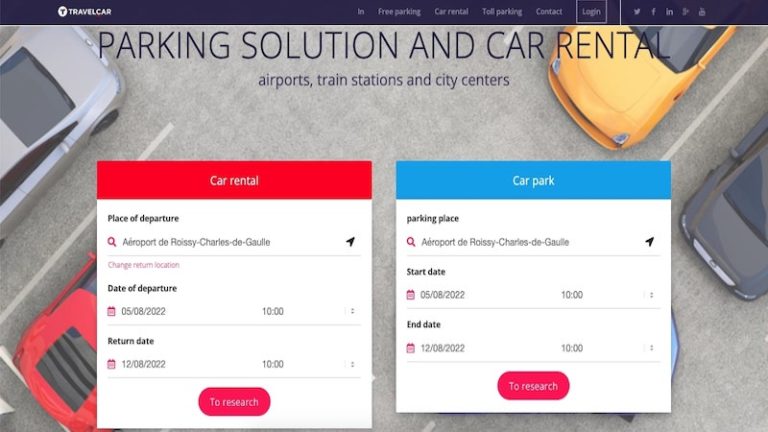The image depicts a comprehensive parking and car rental informational map, primarily aimed at travelers. The title "Travel Car" is prominently displayed, with a navigation section on the side. The map features various parking and car rental options with icons and labels, including "Free Parking," "Car Rental," "Toll Parking," "Contract," "Login," and links to social media. A main heading titled "Parking Solutions and Car Rental" lists key locations such as airports, train stations, and city centers.

In the center of the map, there are two highlighted boxes: one red-labeled box titled "Car Rental" and another blue-labeled box titled "Car Park." The car rental section outlines details for renting a car, including fields for entering the place of departure (e.g., airport or Roissy Charles de Gaulle in France), departure date (August 5, 2022), return date (August 12, 2022), and time (10 a.m. for both departure and return). A red "Search" button is provided for initiating the car rental search.

The parking section beneath it provides information about airport parking at Roissy Charles de Gaulle, also detailing the same departure and return dates and times. Below these sections, there is an aerial photograph showing a car park with vehicles in varying colors—gray, gold, red, silver, and a partial view of a blue car. The parking lot itself is gray with clearly marked white parking space lines. The overall layout is user-friendly, aimed to facilitate easy navigation and planning for travelers.